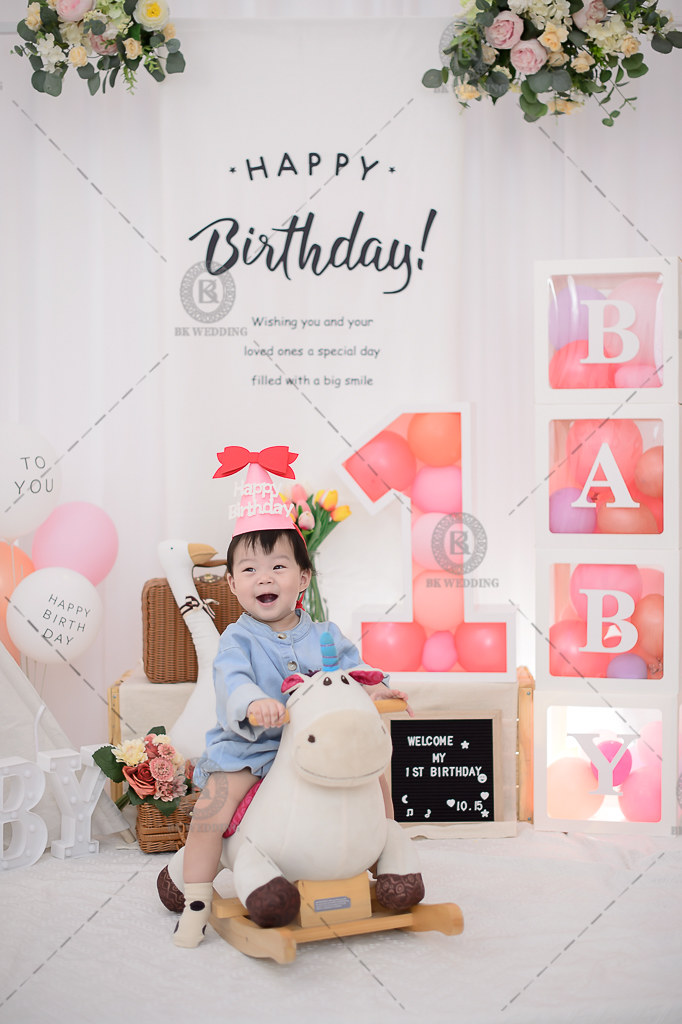The image is a detailed stock photograph designed as a birthday greeting card. Dominating the scene is a smiling toddler sitting on a large, plush, fat unicorn rocker. The child, dressed in a blue dress with buttons, is donning a pink conical birthday hat adorned with a bow on top that reads "Happy Birthday." Behind the child, the background is a pinkish off-white hue, embellished with bouquets of flowers in the upper left and right corners. The central portion of the card features a block and script font text that says "Happy Birthday," along with additional wishes below that read, "Wishing you and your loved ones a special day filled with a big smile." The setting further expresses the birthday theme with a sign that reads, "Welcome My First Birthday," and balloons to the left inscribed with "Happy Birthday." The entire perimeter of the image is marked by a watermark, "BK Wedding," within a gray circle featuring a "B" in the center. The floor beneath the unicorn rocker appears to be white, potentially carpeted, and scattered with more flowers and various other objects.